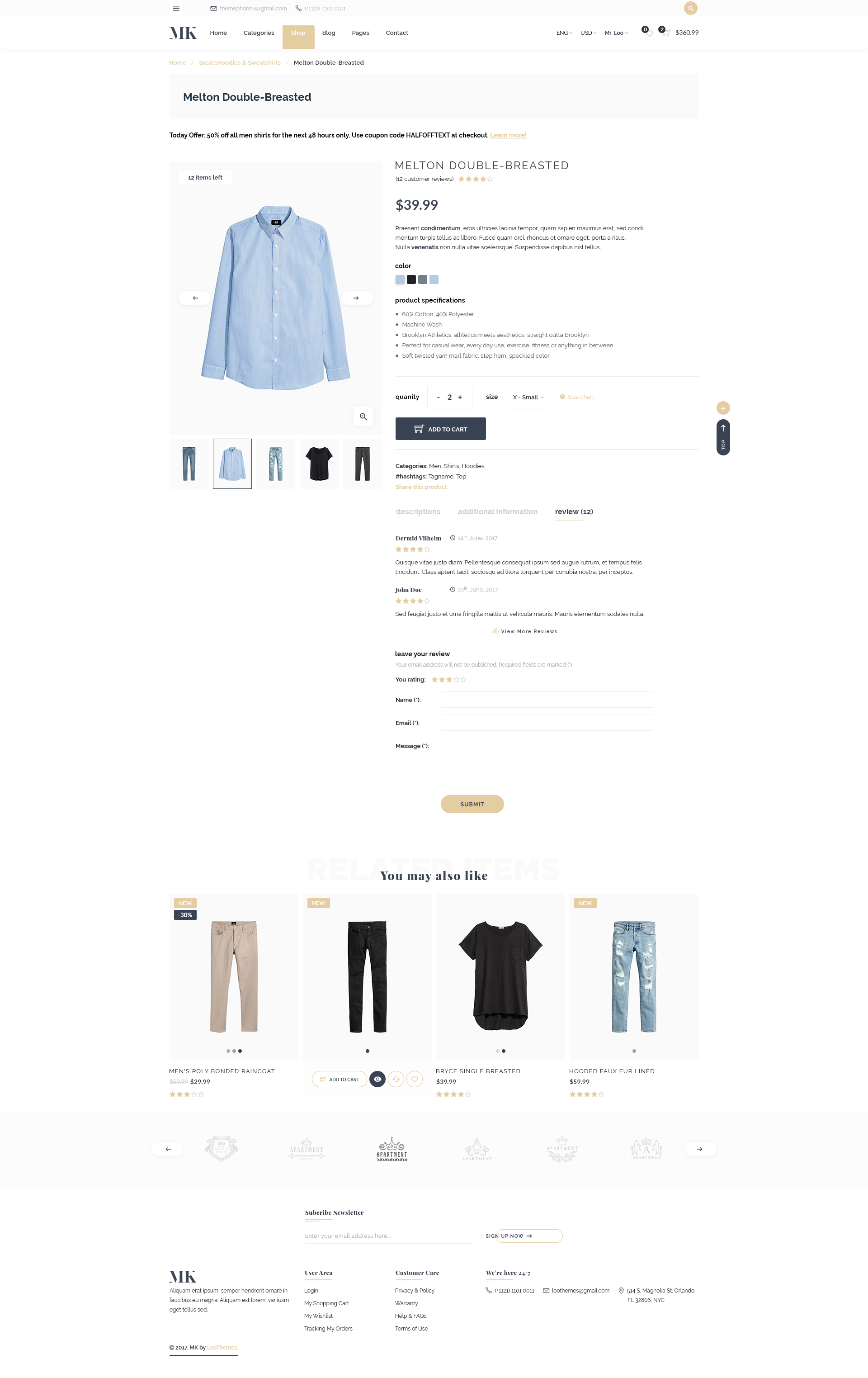The image is a screenshot of a website, featuring a clean layout and a slightly colorful header. At the very top, it displays a simple graphic along with contact information, including an email address and phone number. The primary navigation menu follows, which includes links to "Home," "Categories," "Shop," "Blog," "Pages," and "Contact." Notably, the "Shop" link is highlighted with a tan background and white text, standing out from the others that are in black text on a white background.

Below the navigation menu, the page features breadcrumbs that read "Home > Hoodies and Sweatshirts," displayed in light tan text, making them somewhat difficult to read. Immediately below is a prominent heading in black text that reads "Melt and Double Breasted."

A banner section follows, boldly proclaiming "Melt and Double Breasted" again, accompanied by a promotional message: "Today's offer: 50% off all men's shirts for the next 48 hours only. Use coupon HALF OFF at checkout."

The next section features a gray background with an image of a blue button-down shirt. Above the product image, it states that only 12 items are left. The product name "Melt and Double Breasted" is displayed again with the price marked at $39.99. There are four different color options available for selection.

Further down, the product's specifics are outlined, including options for Quantity, Size, and an "Add to Cart" button. The categories listed are "Men’s Shirts" and "Hoodies," with tags such as "Hashtag," "Tag Name," and "Top."

At the bottom of the page, there is a section for customer reviews where users can leave a rating, name, email, and message. A "Submit" button allows users to post their reviews. Finally, additional clothing items are showcased, providing more shopping options.